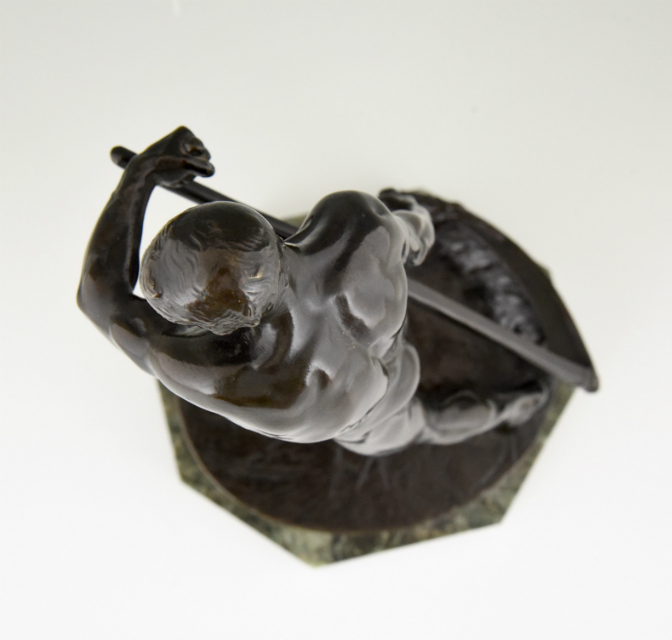The image depicts a high-angle photograph, likely taken indoors, showing a glossy, black-colored statue which appears to be made of metal or potentially marble. The statue, viewed from above, features a naked man standing on a base that is either a hexagon or pentagon or almost circular. The background of the photo transitions from gray at the top to nearly white at the bottom, devoid of any borders. The man in the statue is turned slightly, looking down and to the left, making his facial features and eyes not visible. His left arm, bent at the elbow, holds onto a rod or a long sword above his head, while his right arm hangs down by his side. The feet of the statue are firmly placed on the glossy base, anchored at different points, giving it a balanced stance. The photograph captures the intricate details and reflective quality of the statue, highlighting its glossy finish against the contrasting pale background.